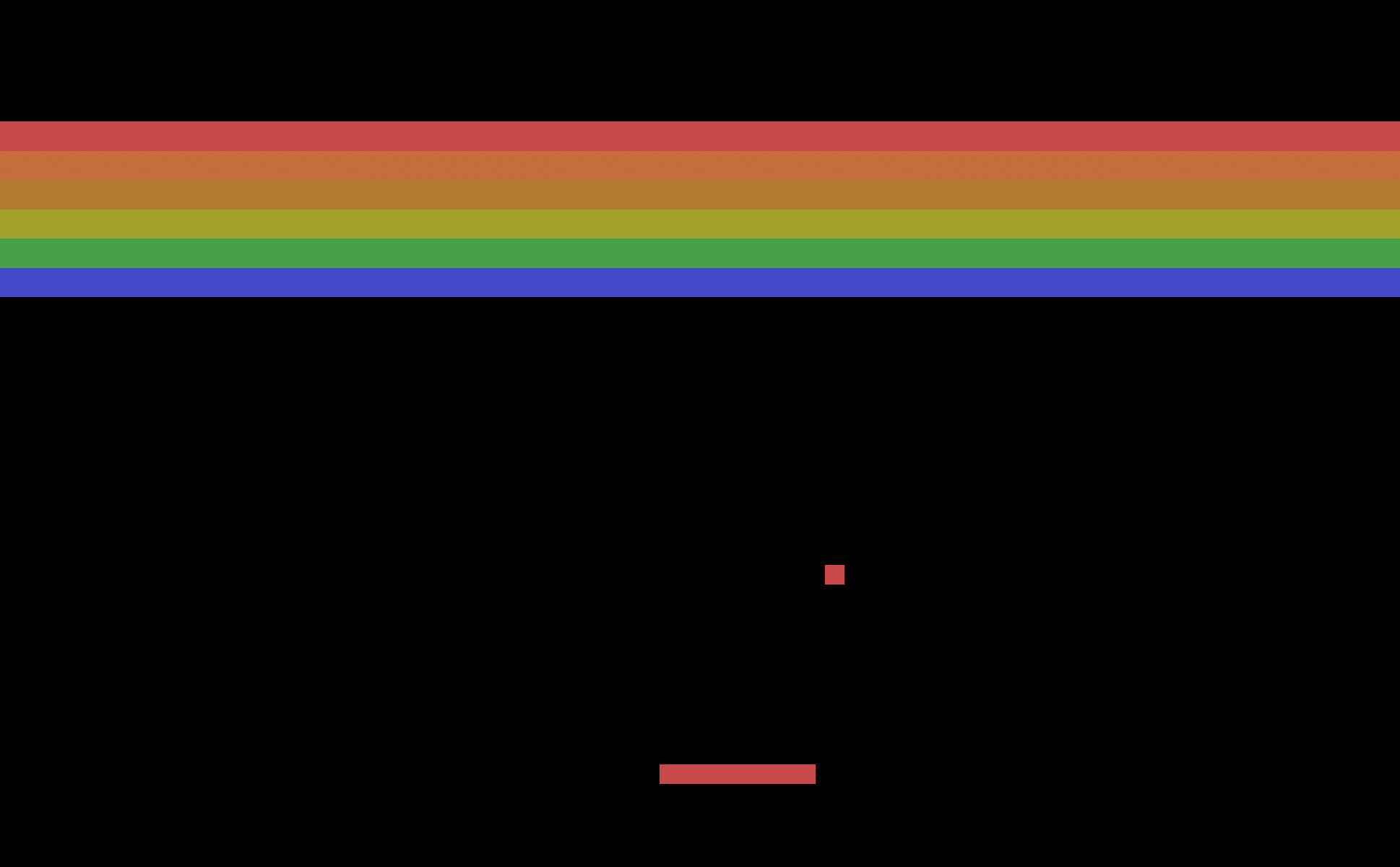This striking photograph features a solid black background, providing a vivid contrast to a prominently displayed horizontal rainbow stripe collection that spans the entire width of the image. From top to bottom, the vibrant stripes are perfectly uniform in thickness, starting with a bold red stripe, followed by an orange stripe, a goldish-orange stripe, a bright yellow stripe, a fresh green stripe, and, finally, a deep blue stripe. At the very bottom of the image, below the rainbow, stands a thin red rectangular bar, accompanied just above by a small red square, reminiscent of the classic elements found in the game Brick Breaker.